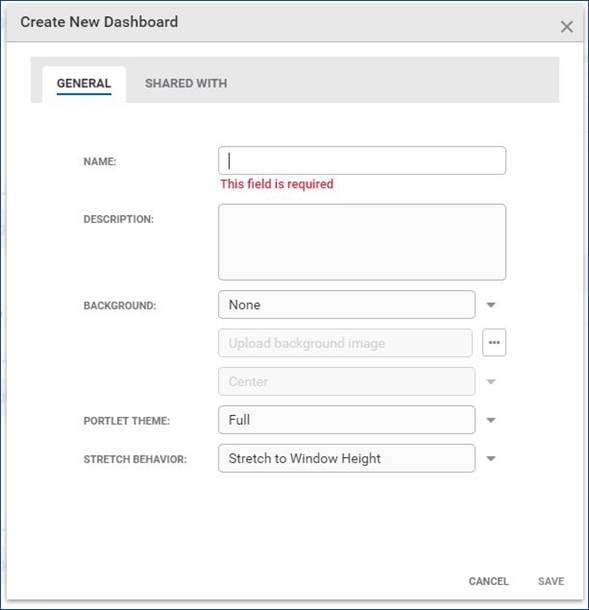The image depicts a user interface for creating a new dashboard. At the top left, there is a title in black text, "Create New Dashboard". The navigation bar below it is colored light gray and contains two tabs: "General," which is selected and highlighted with a teal underline, and "Shared With," which is grayed out and not selected. 

Below the navigation bar, there is a form beginning with a selection box for the dashboard name, indicated by the label "Name:" followed by a cursor icon implying text entry, although no text is present. A red warning message, "This tool is required," appears beneath the entry box.

Further down is a larger description box, which is currently empty. Below this, there are controls for background settings. The "Background" label is followed by a drop-down menu set to "None". Below this, there are grayed-out options for "Upload Background Image" and "Center," along with an upload button featuring a three-dot icon on the right.

The "Portlet Theme" section follows, presenting a filled selection box. At the bottom, "Stretch Behavior" is set to "Stretch to Window Height," which is selected. Finally, at the very bottom right, there are two buttons, "Cancel" and "Save," both rendered in gray, indicating they are currently inactive.